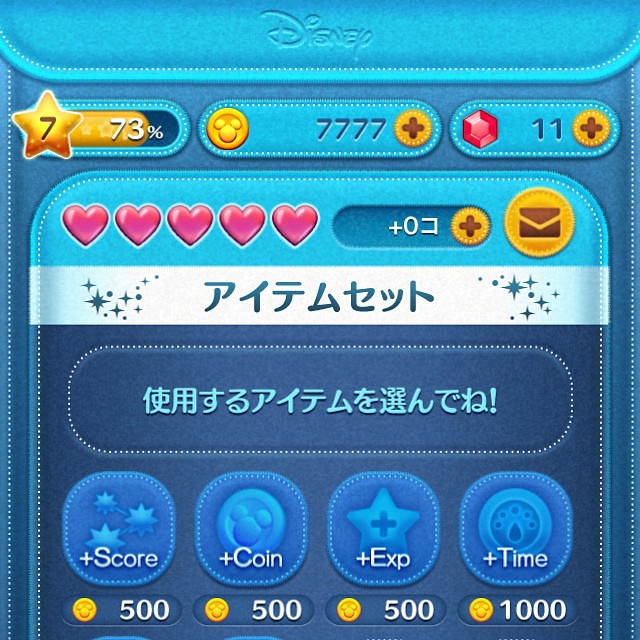The image is a detailed screenshot of a mobile game interface with a primarily dark blue, leather-like background with white stitching accents reminiscent of teal leather. At the top of the screen, "Disney" is prominently displayed in the recognizable Disney font. In the top left corner, there is a yellow star partially enclosing the number 7, which is accompanied by a gold progress bar extending to the right, showing 73%. Adjacent to this star in the center of the screen is a circular icon featuring the number 7777, also accompanied by a plus sign. To its right is a red octagon-shaped gem labeled with the number 11 and a yellow plus symbol.

Beneath these elements, there are five red hearts indicating lives or health, positioned on the left side of the screen. The right side features a brown message log within a yellow circular background. 

At the bottom of the screen, there are four horizontal bars labeled as score, coin, experience, and time, each with a corresponding value of 500, except for time which is valued at 1000. These values are displayed next to small Mickey Mouse symbols, presenting the shape of Mickey’s face and ears, underscoring the game’s Disney theme. There are additional Japanese characters visible in various parts of the interface, enhancing the thematic authenticity and user experience.